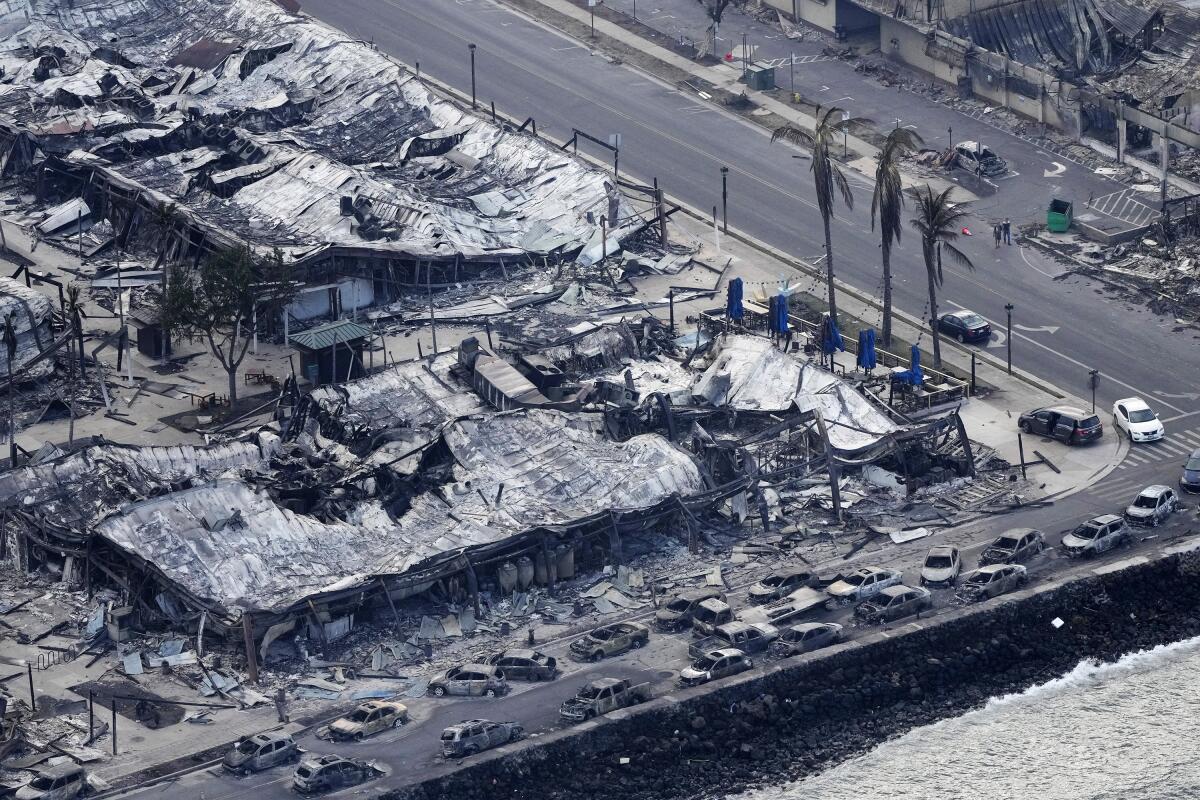The black and white photo dramatically captures the aftermath of a major disaster in what appears to be a coastal city, potentially in Hawaii or Miami, marked by utter devastation. Prominent in the foreground are palm trees, surprisingly still standing amidst the wreckage. Centered in the image are buildings that have been completely destroyed, their roofs gone, and structures seemingly charred and flattened. The destruction extends to the roads, littered with cars burned out and demolished, aligning from the bottom left corner diagonally upwards. Shades of black, white, and gray dominate the scene, with glimpses of blues and greens suggesting remnants of what was once vibrant. A road with faded directions cuts through the chaos, highlighting the incongruity between the usual and the catastrophic. The photo starkly shows a complete breakdown of the urban landscape, underscored by a backdrop of severe weather damage or possible wildfire, leaving an indelible mark of horror and desolation.